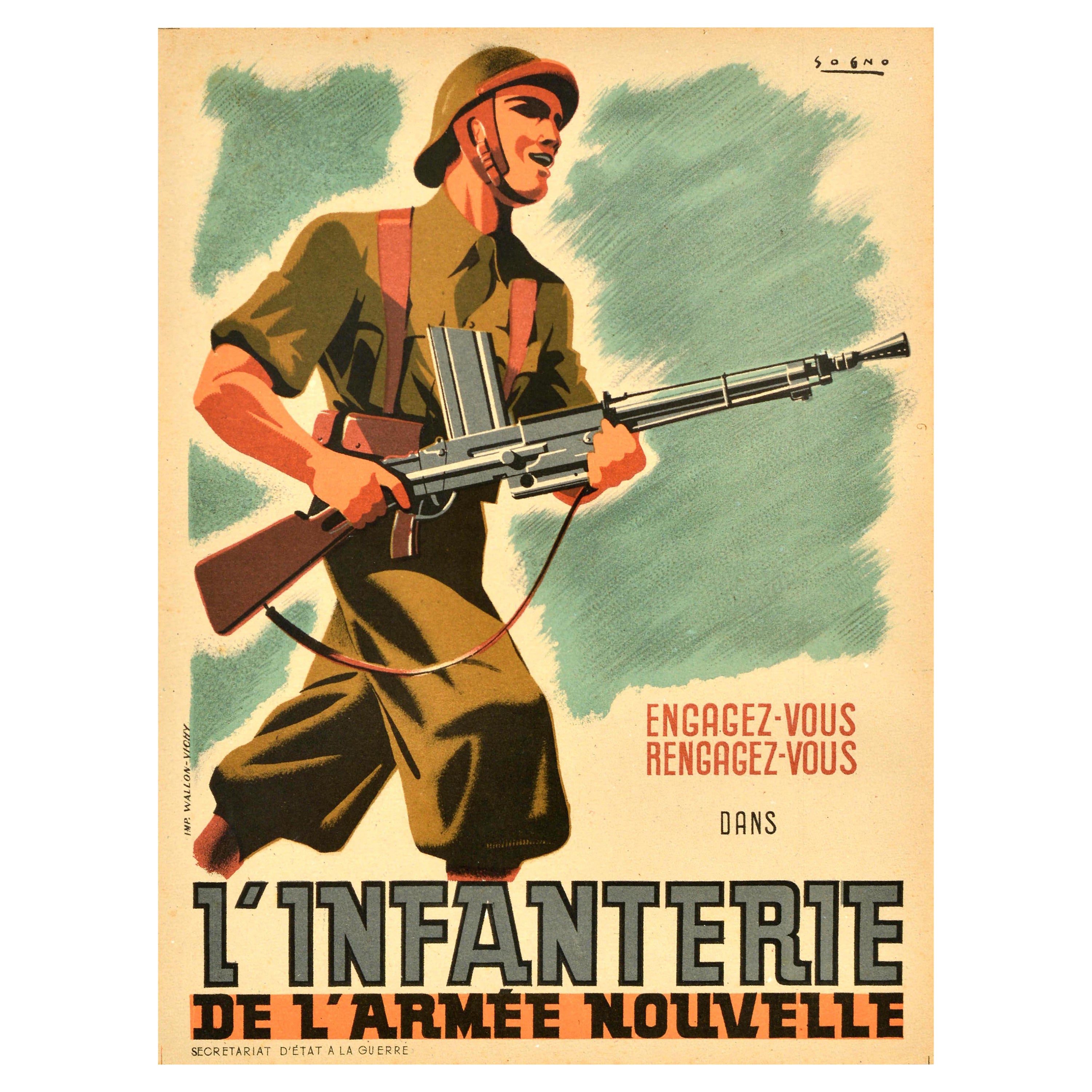This detailed and cohesive caption fuses the elements from all three descriptions:

This poster, likely from World War I, features a soldier in a monochromatic schematic, predominantly green and brown. He dons a green uniform with brown leather straps crisscrossing his chest, a green helmet with matching brown straps and rim, and baggy green leggings. The soldier, who holds a rifle with a banana clip facing up, stares solemnly into the distance, his facial features obscured in shadow, giving him a stern and enigmatic presence. Surrounding him is text in what appears to be French. Prominently, red text reads "Engagez Vous," likely a call to action, while the bottom of the poster declares "L'infanterie de l'armée nouvelle" in bold letters, identifying it as an infantry recruitment piece. The poster's background includes blue splotches, contrasting with the solemn figure and adding an element of depth to the design.